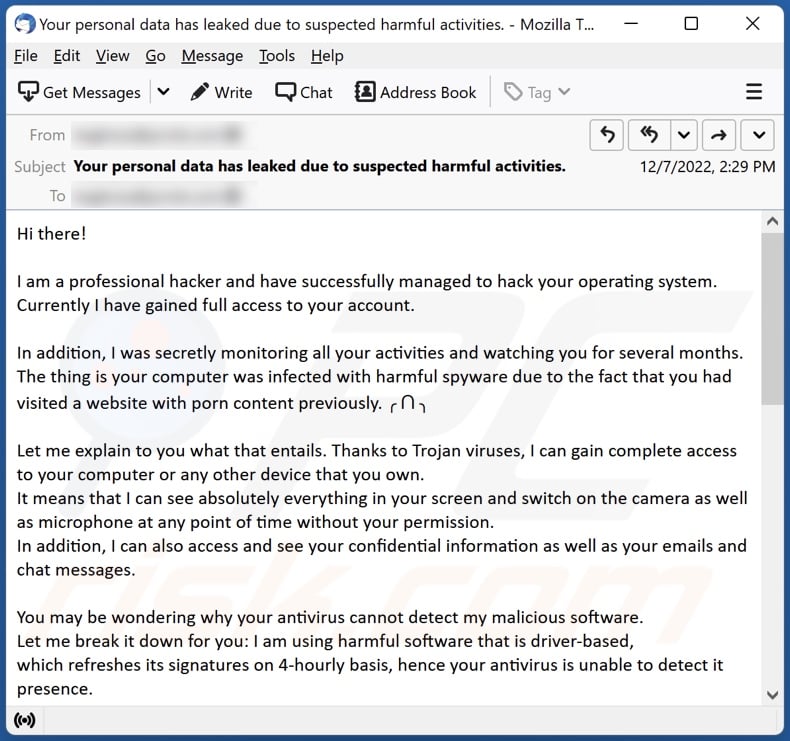This image displays a screenshot of a Mozilla email inbox, showcasing a threatening phishing email. Highlighted by a thin blue border, the email's subject line reads "Your personal data has leaked due to suspected harmful activities," and a timestamp of "12-7-2022 at 2:29 p.m." is visible. The "From" and "To" fields are blacked out, maintaining privacy. The interface includes standard Mozilla email client tools like 'File,' 'Edit,' 'View,' 'Go,' 'Message,' and 'Tools,' with icons below for 'Get Messages,' 'Write,' 'Chat,' and 'Address Book.'

The body of the email contains a disturbing message from a self-proclaimed "professional hacker," claiming to have hacked the recipient's operating system and monitored their activities for several months. The hacker asserts that the computer was infected with spyware due to visits to pornographic websites. The email warns of complete access to the recipient's devices, including control over the camera and microphone, and detailed monitoring of their confidential information and communications. The message attempts to explain why antivirus software failed to detect the malicious software, attributing it to advanced, driver-based malware that refreshes its signatures every four hours. This appears to be a typical spam email designed to scam recipients into believing their data and privacy are compromised.